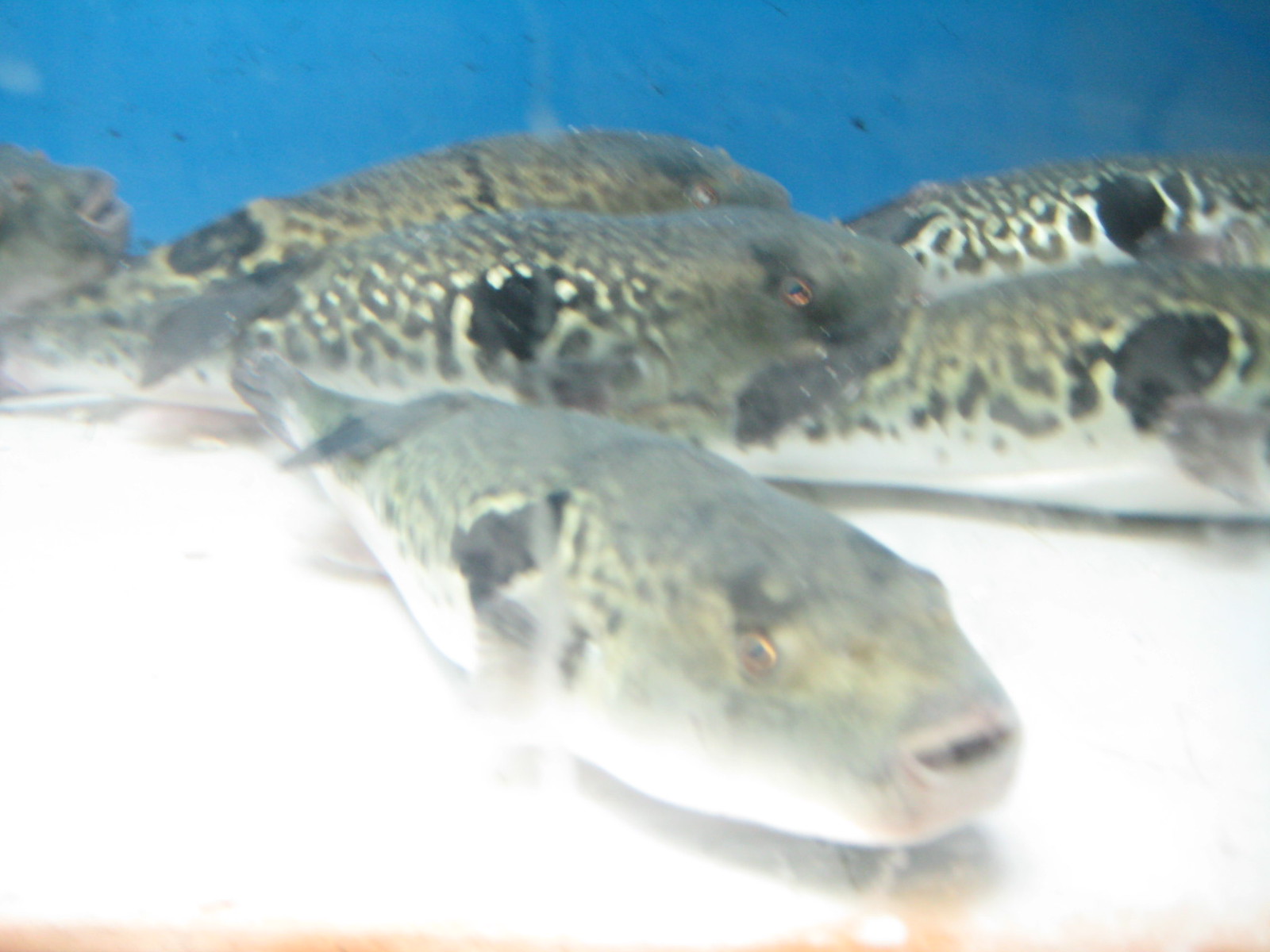The image depicts a slightly out-of-focus photograph of six medium-sized fish, appearing to be of the same species, resting near the bottom of what seems to be an aquarium. The aquarium wall is a clear turquoise blue, providing a serene background. The floor or base of the tank is a light, almost white color with a subtle orange film along its border. The fish are arranged with three visible in the middle, another fish peeking from the left, and parts of two more fish on the right. These fish have a distinctive appearance: their backs are speckled in shades of dark and light brown, greenish in hue with intricate patterns resembling circular stripes and dots. Each fish bears a dark eye spot on its side and dark tails, with pale underbellies, and notable orange accents around their eyes, which appear large and expressive. Their small, seemingly smiling mouths add a subtle charm to their appearance. The overall scene feels slightly psychedelic due to the fish's patterns and the blurred quality of the photograph.